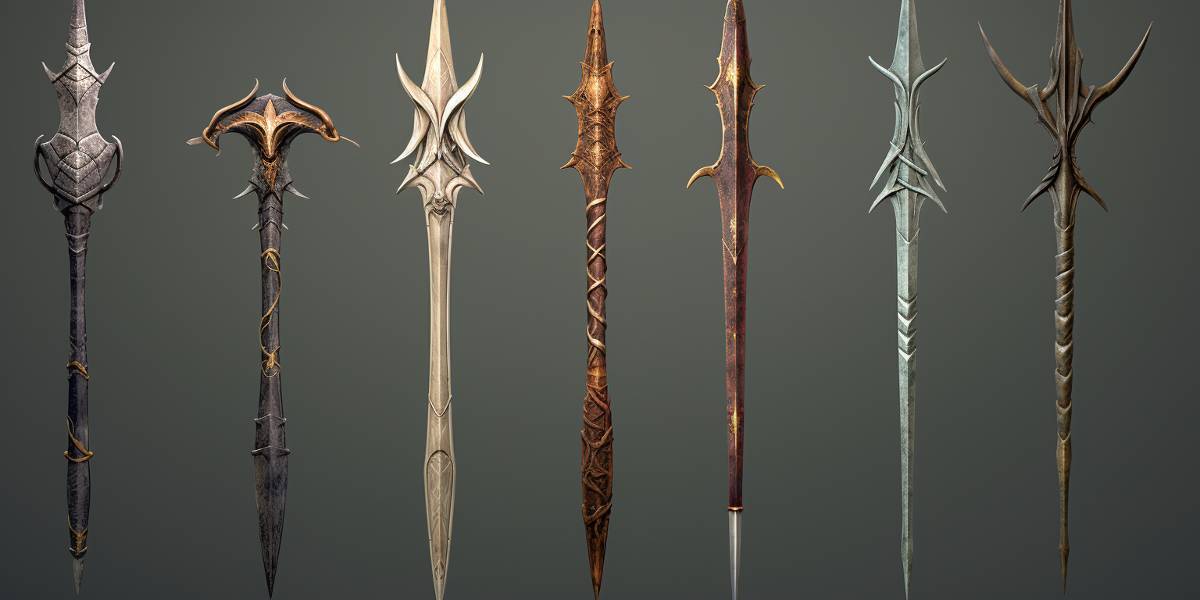The image displays seven vertically-aligned weapons against a charcoal gray background, ranging from axes to intricately designed daggers and staffs. The entire setting is illuminated brightly, providing clear visibility of each weapon's unique features. Starting from the left, the first weapon is a staff with a gray top and a black shaft running down to its base. The second weapon is predominantly black, features subtle yellow accents, and has a pointed end. Next, there is a lighter-colored, silver-toned metal weapon, followed by a copper-colored staff adorned with rope-like strands. Moving right, the fourth weapon is a sleek brown staff with a sharp needle-pointed end. Adjacent to it is another silver-toned metal staff distinguished by its triangular edges. Finally, on the far right, there is a distinctively brown staff featuring a design that resembles devil horns. Each piece appears to be very ornate, with handles that showcase intricate carvings and embellishments. The variety of the materials, which include silver, copper, black metal, and more, highlights the diverse craftsmanship of these historical-looking weapons.